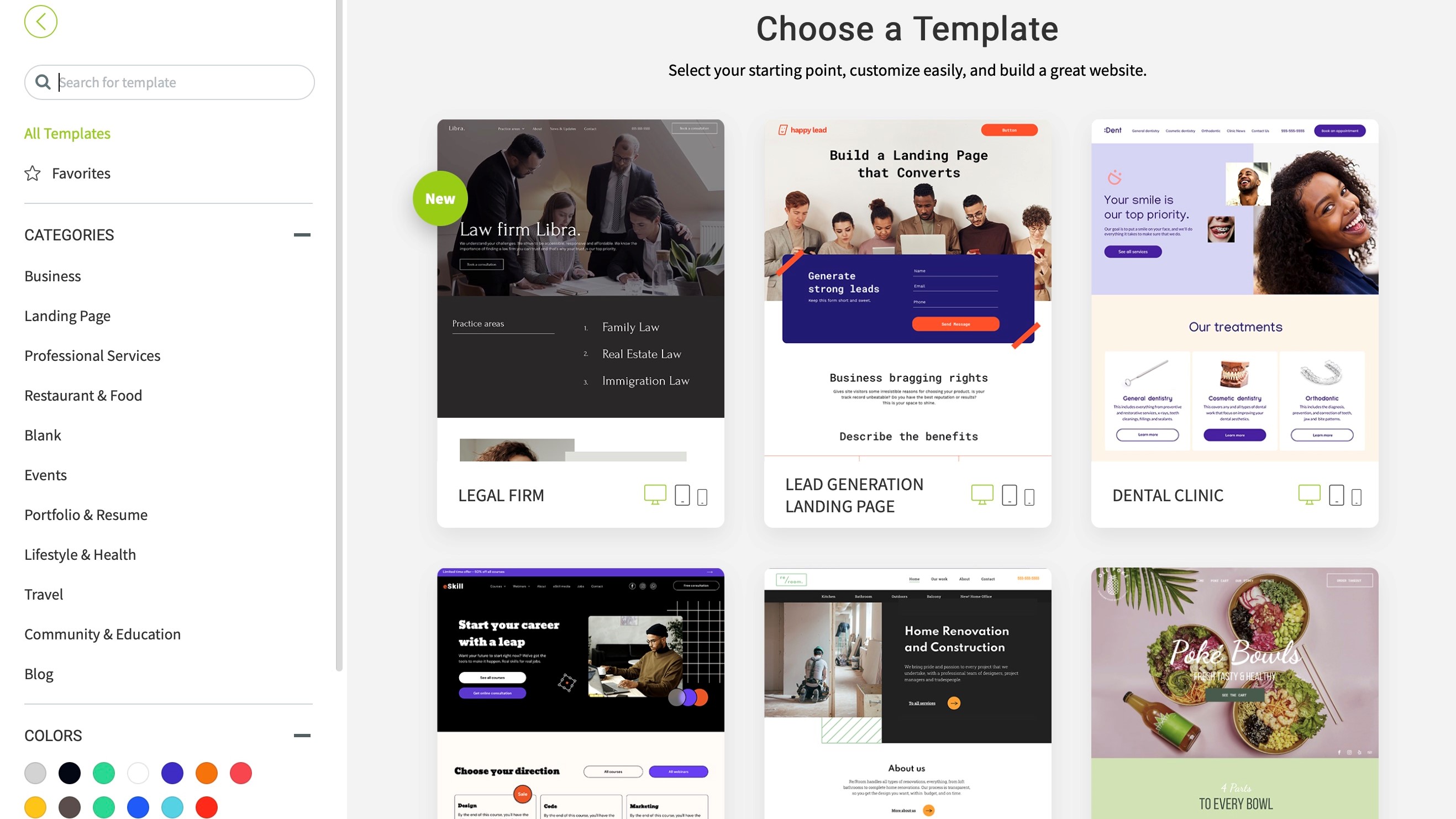The image depicts a screen capture of an online application page designed for selecting website templates. The background of the screen is a very light beige or white color, providing a clean and minimalist appearance. On the left side of the screen, a vertical frame features a white background. 

At the top of this vertical frame is a search bar, facilitating easy navigation. Directly below the search bar, the text "All Templates" is displayed in green, indicating the section's content. Under this heading, there are several listings of available templates, showcasing a range of options. Towards the bottom left of this frame, a series of color selections is visible. These colors are presented in round circular frames, likely for easy color theme customization.

The remainder of the screen, occupying the right side of the image, showcases six distinct website templates. At the top of this section, a heading in black text reads, "Choose a template. Select your starting point. Customize easily and build a great website." This directive guides users through the initial steps of the website creation process. 

The templates are organized into two rows, with three templates in each row, offering a visually accessible layout for comparison and selection. This structured presentation allows users to effortlessly browse and select their preferred template to begin customizing their website.